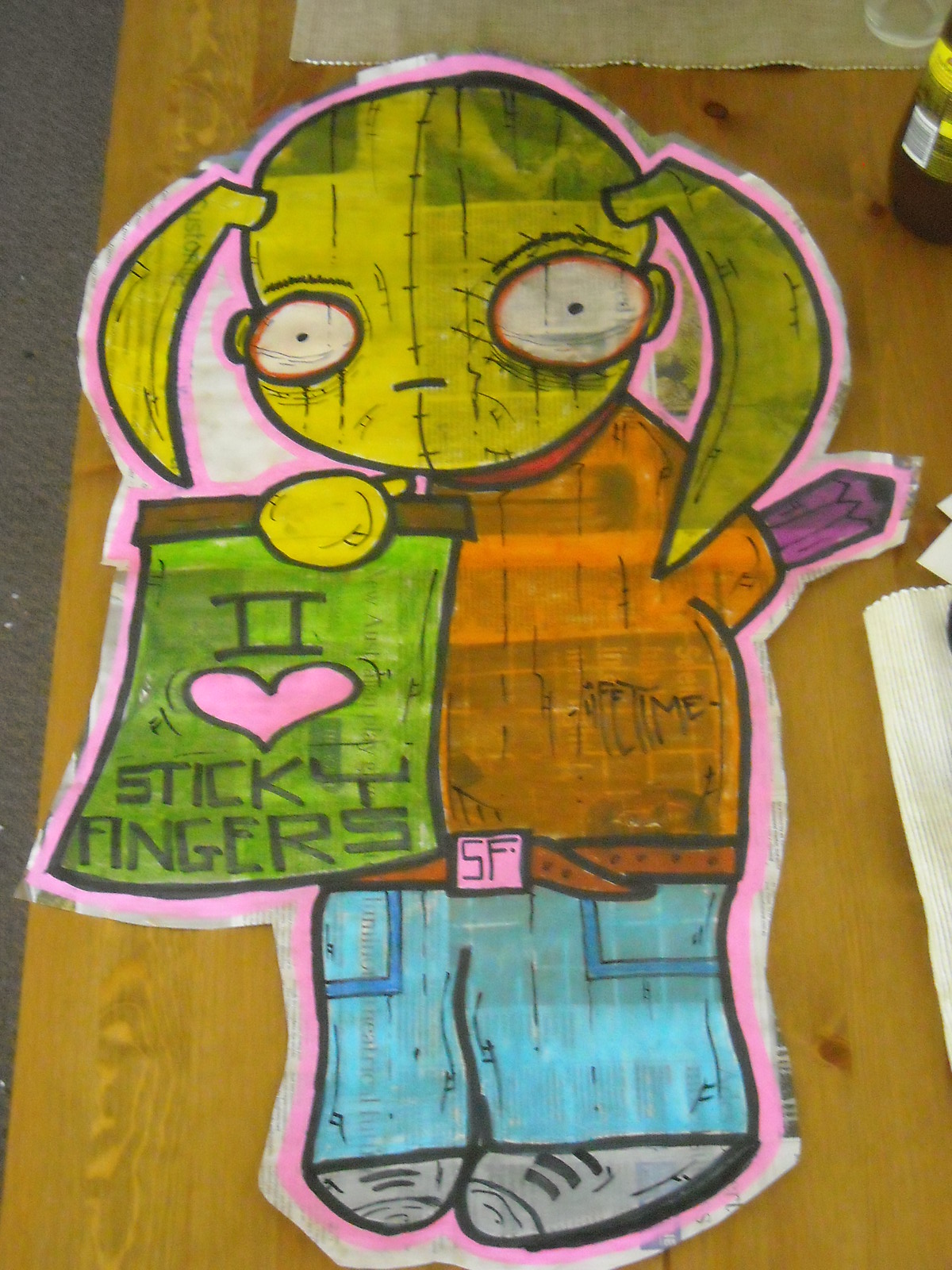In the image, a colorful hand-drawn character is displayed on a piece of paper, laid out on a light brown wooden table. To the top right of the scene, a bottle of iced tea, likely from a vending machine, partially obscures the view. There are also cloth or paper placemats scattered around, adding texture to the background. The main focus of the illustration is a whimsical cow-like creature with large ears, a round yellow head, and a minimalist face featuring slit-like nostrils and expressive eyes outlined in red. The creature is dressed in an orange shirt and blue pants, sporting gray tennis shoes. An orange belt with a pink SF buckle cinches its waist. Notably, its right arm is depicted as a purple pencil. The creature grasps a green parchment that reads "I ♥ sticky fingers" in black print, with a pink heart accentuating the message. The artwork is meticulously outlined in pink, making the character stand out against the white paper background. The setting appears to be a cozy indoor environment, perhaps a kitchen or coffee table, with a sliver of carpet visible on the left side of the image.